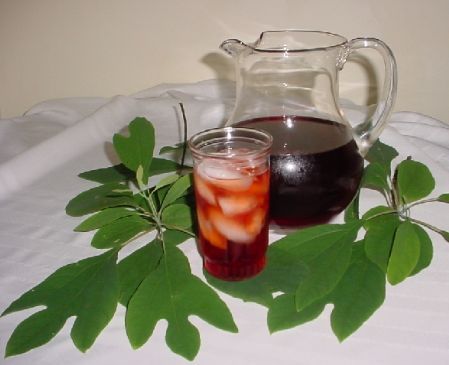The image depicts a clear glass pitcher filled with a dark reddish liquid, possibly juice or tea, suggesting the color of cranberry juice or cherry compote, with hues varying from reddish to purple. The pitcher, which is rounded at the bottom and features a large handle, is set on a white tablecloth-covered surface, likely a tray. Accompanying the pitcher is a tall glass containing the same beverage over ice, showcasing more of the reddish color in contrast to the pitcher. Adjacent to these items are sprigs of wide green leaves, arranged decoratively on the tablecloth. The background of the image consists of a white-washed wall, enhancing the clean, minimalistic aesthetic of the setup. This arrangement, likely intended for social media or a blog, hints at a recipe or a lifestyle post.